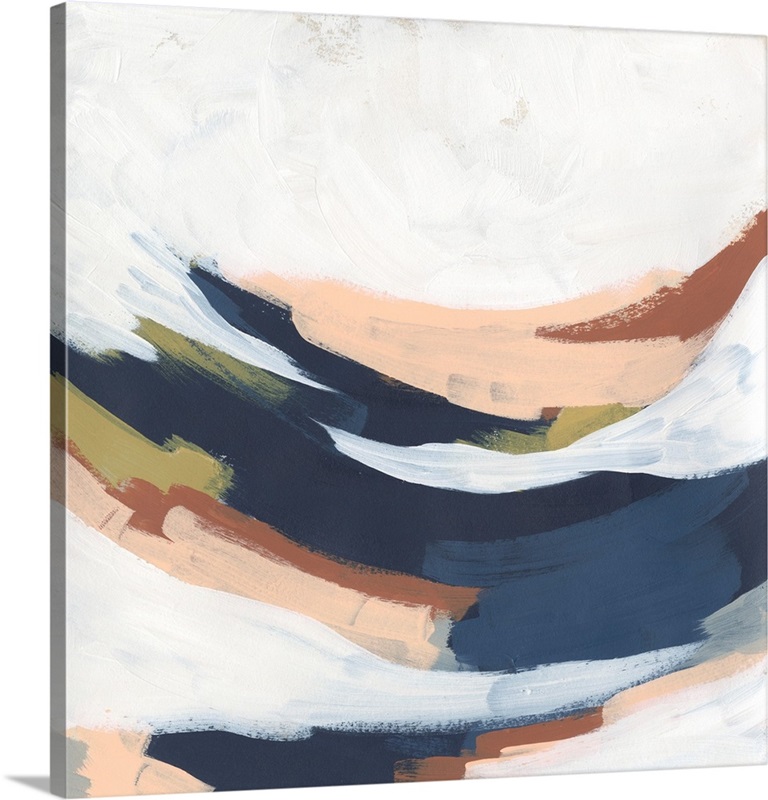This image depicts an abstract painting on a square, thick-framed canvas, encompassing modern art. Predominantly white in the background, the painting features a mix of tan and bluish-gray hues. Big, sweeping brushstrokes create a sense of motion and depth. Beige, brown, and dark blue streaks dominate the composition, with the blue tones concentrating in the middle-bottom section. Notable are the three arch-like streaks that run across the image, adding an intricate layer to the otherwise freeform brushstroke patterns. The beige and brown brushstrokes contribute to the earthy palette, intermingled with subtle green hints. The painting’s abstract nature is underscored by broad, colorful bands and pointed shapes reminiscent of turned-up leaves, providing a textured, layered aesthetic. The image wraps around the edges of the canvas, enhancing its three-dimensional appearance.